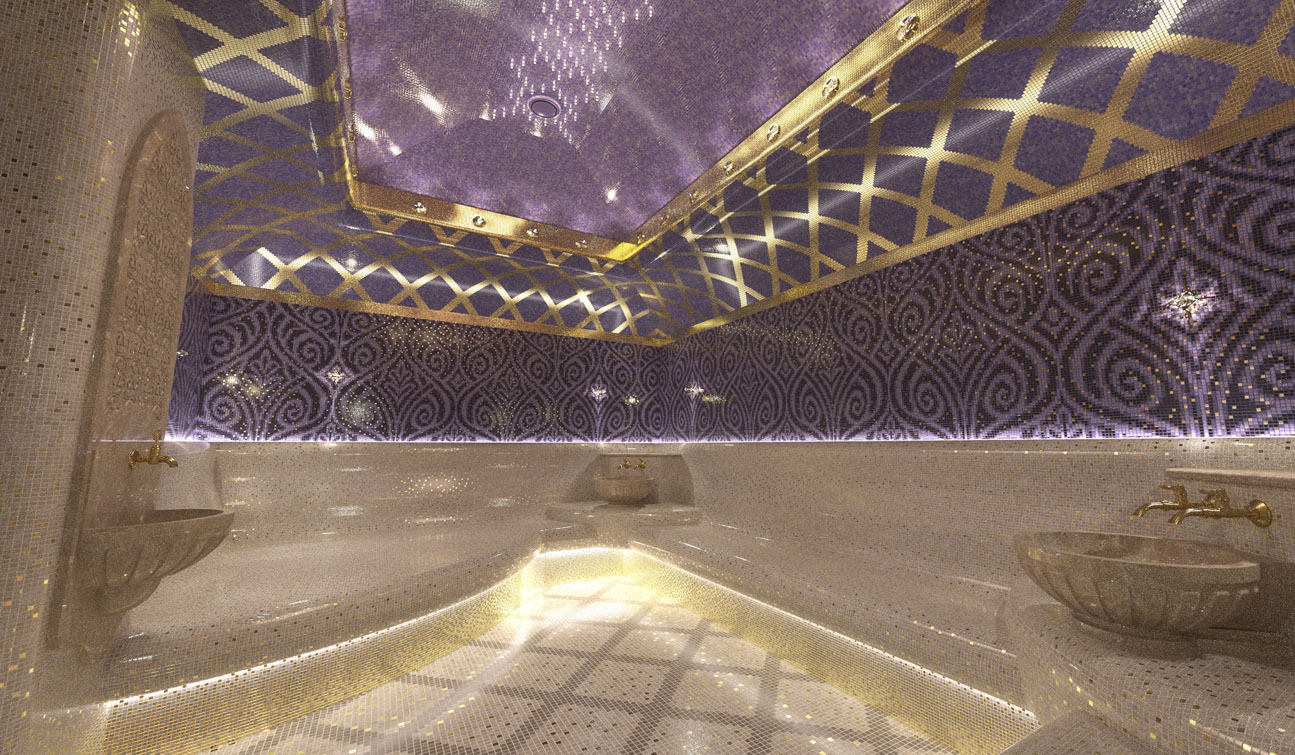The image captures a lavish bathroom, reminiscent of those found in a Vegas casino, featuring opulent Middle Eastern architectural elements. The ceiling is predominantly purple, adorned with intricate gold X and diamond patterns, further complemented by gold trim. It showcases three tan ceramic sinks, each equipped with dual gold faucets, harmoniously matching the sink's design. The sinks are positioned apart across the space, one on the left within a curved wall, another centered, and the third on the right. 

The flooring consists of tan speckled tiles with gray grout lines, enhancing the room's luxurious feel. The lower portion of the image reveals a recessed seating area with a long bench stretching from left to right, covered in small whitish and gold-toned tiles. This area mirrors the elegance of the decor with its scalloped-shaped sinks under gold faucets, extending the theme of grandeur.

Above the seating area, the wall features purple tiles adorned with black tiles forming intricate leaf, flower, and spiral designs. Highlighting its recessed nature, the wall is bordered with gold tiles featuring diamond shapes, culminating in a purple-tiled ceiling encircled by a band of gold trim and finished with subtle lighting. The combination of rich purples and shimmering golds throughout the space evokes a sophisticated and exotic ambiance.